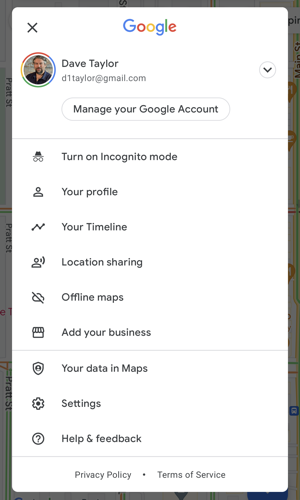This image depicts a screenshot of a Google account management page, presumably accessed via a web browser or a mobile app. The screenshot is enclosed within a thin, slightly curved border, giving the impression of a layered interface with a shadowed, almost grey backdrop.

At the top center of the screen, a multi-coloured Google logo stands out against a white background. On the left-hand side of the banner is a small 'X' icon, and to its right is a circular avatar showing a man's head with light skin and short hair, wearing a black shirt. This avatar is labeled "Dave Taylor," along with his email address, "davetaylor@gmail.com." To the right of the avatar, a down arrow indicates a dropdown menu for additional options.

Below the banner is a horizontally aligned, curved rectangle button with the text "Manage your Google Account," hinting at additional account management features. Directly under this button is a horizontal dividing line, separating the account management button from the subsequent list of options.

The list, running vertically down the screen, consists of several labels, each accompanied by small, black-and-white icons on their left. The labels are as follows: "Turn on Incognito mode," "Your profile," "Your timeline," "Location sharing," "Offline maps," "Add your business," "Your data in Maps," "Settings," and "Help & feedback."

At the bottom left corner of the screen, the terms "Privacy Policy" appear, followed by a small dot or separator, and then "Terms of Service" towards the right. These terms are centrally aligned horizontally but positioned on opposite sides of the line, indicative of legal informational links.

Overall, the screenshot captures a comprehensive overview of a Google account management interface, complete with various settings and options tailored to user privacy, profile management, and map-related functionalities.